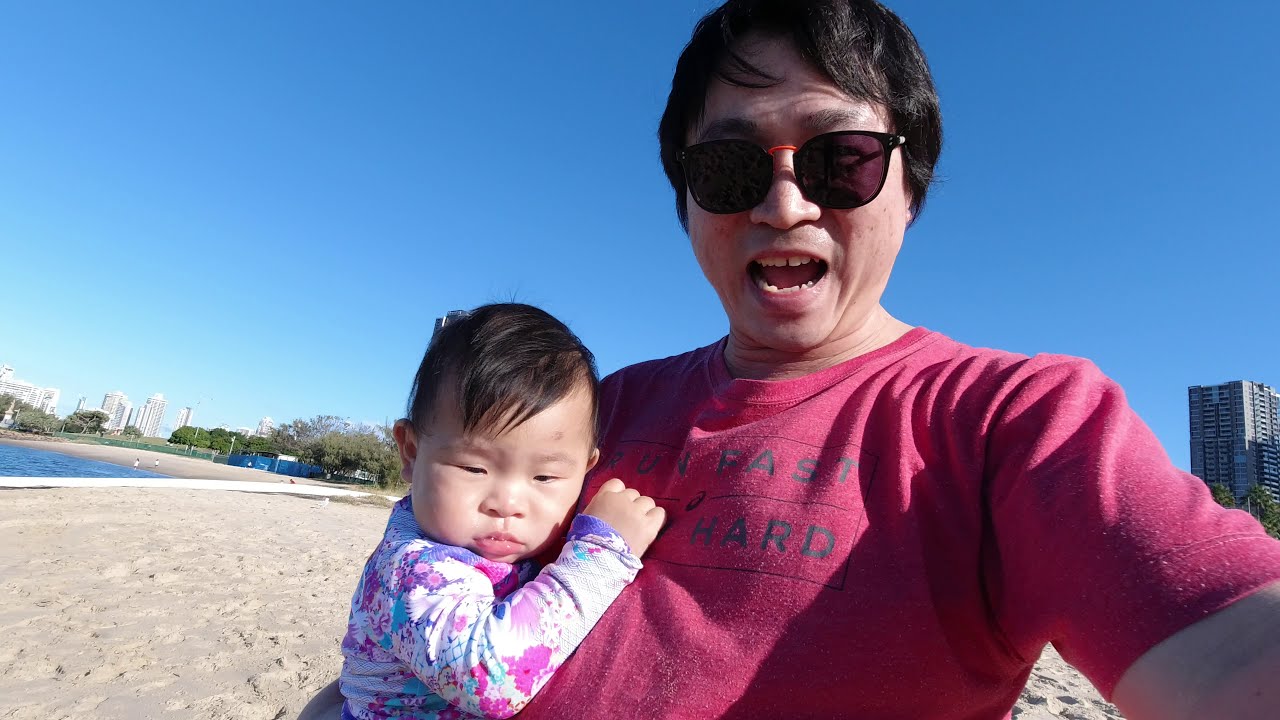In this vibrant outdoor photograph, a lighter-skinned adult with short black hair, outfitted in stylish sunglasses and a red short-sleeved shirt, is captured mid-expression, perhaps engaging playfully or making a funny face. Cradled in the adult's right arm is a young child, likely around six months old, also of lighter complexion with short dark hair, dressed in a charming long-sleeved shirt adorned with white, purple, and pink floral patterns. The scene is set against a picturesque backdrop of a beach area, revealing sandy shores and a body of water, complemented by distant white buildings and verdant green trees. The bright blue sky stretches across the upper portion of the image, bathing the entire scene in plentiful natural daylight. The engaging composition, framed in landscape orientation, showcases an intimate, candid moment between the adult and child, set within a serene and sunlit coastal environment.